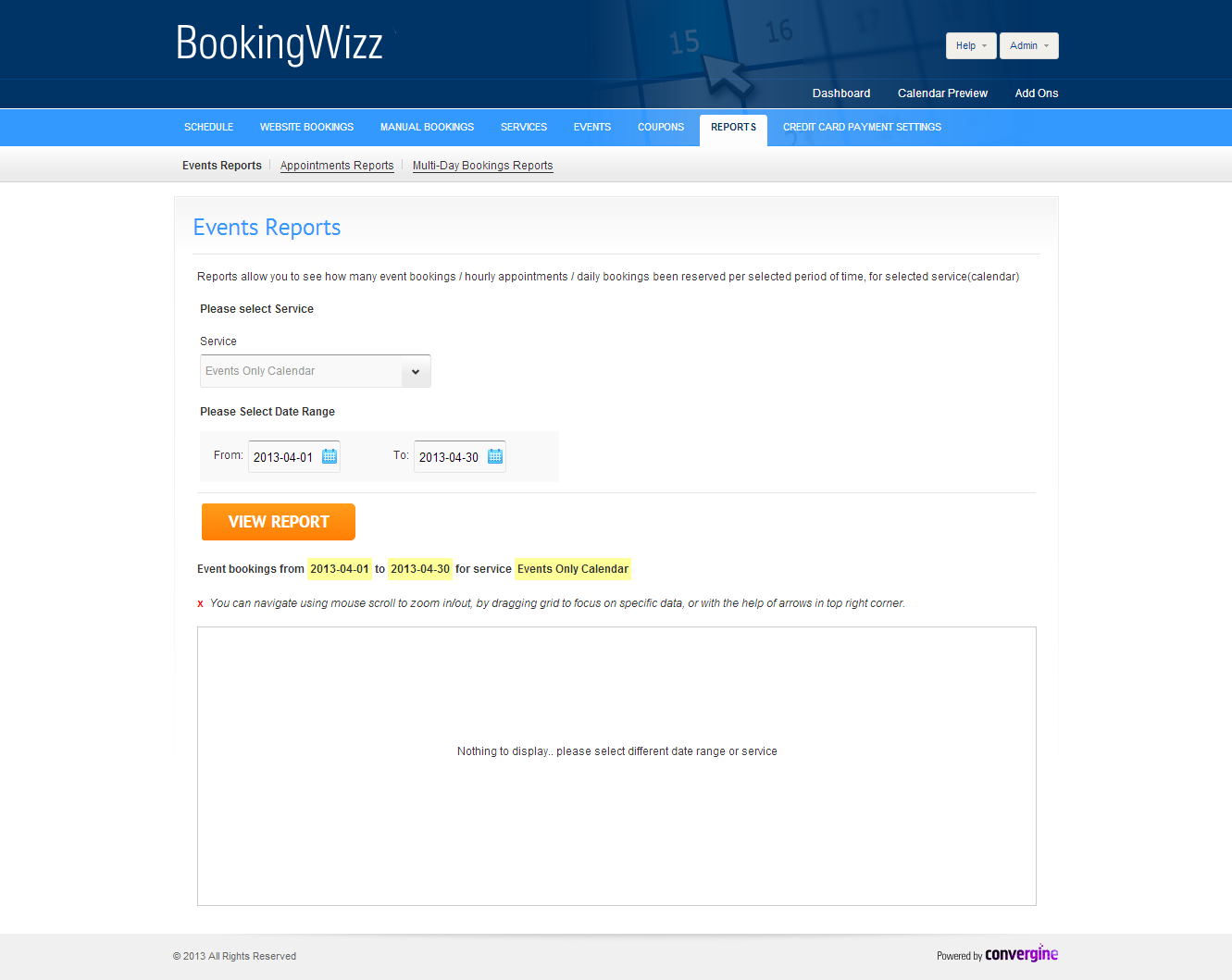This detailed color photograph captures a vibrant and organized interface of a website displayed on a computer or laptop screen. At the very top, a blue banner spans the width of the screen. On the left side of this banner, white text reads "Help," while on the right side, two small white rectangles contain "Admin" and "Help" in black letters.

Directly below this banner, another set of white text is neatly arranged: "Dashboard," "Calendar," "Preview," and "Add-ons." Further down, a smaller horizontal banner lists "Schedule," "Website Booking," "Manual Bookings," "Services," "Events," "Coupons," "Reports" (which is highlighted), and "Credit Card Payment Settings," all in white letters.

Beneath this banner, bold black text labels different sections: "Event Reports," "Appointment Reports" (underscored), and "Multi-Day Booking Reports" (also underscored). 

In a rectangular window below, the headline "Event Reports" is displayed in light blue letters. The explanation underneath, in black text, states: "Reports allow you to see how many event bookings/hourly appointments/daily bookings have been reserved per selected period of time, for selected service calendar." Following this, prompts are given: "Please select a service" with a dropdown box, "Please select a date range," and a button labeled "View Report." Below these prompts, there is a dedicated window area for viewing the selected report.

The overall layout is clear and functional, designed to help users navigate through various administrative tools and reporting features efficiently.